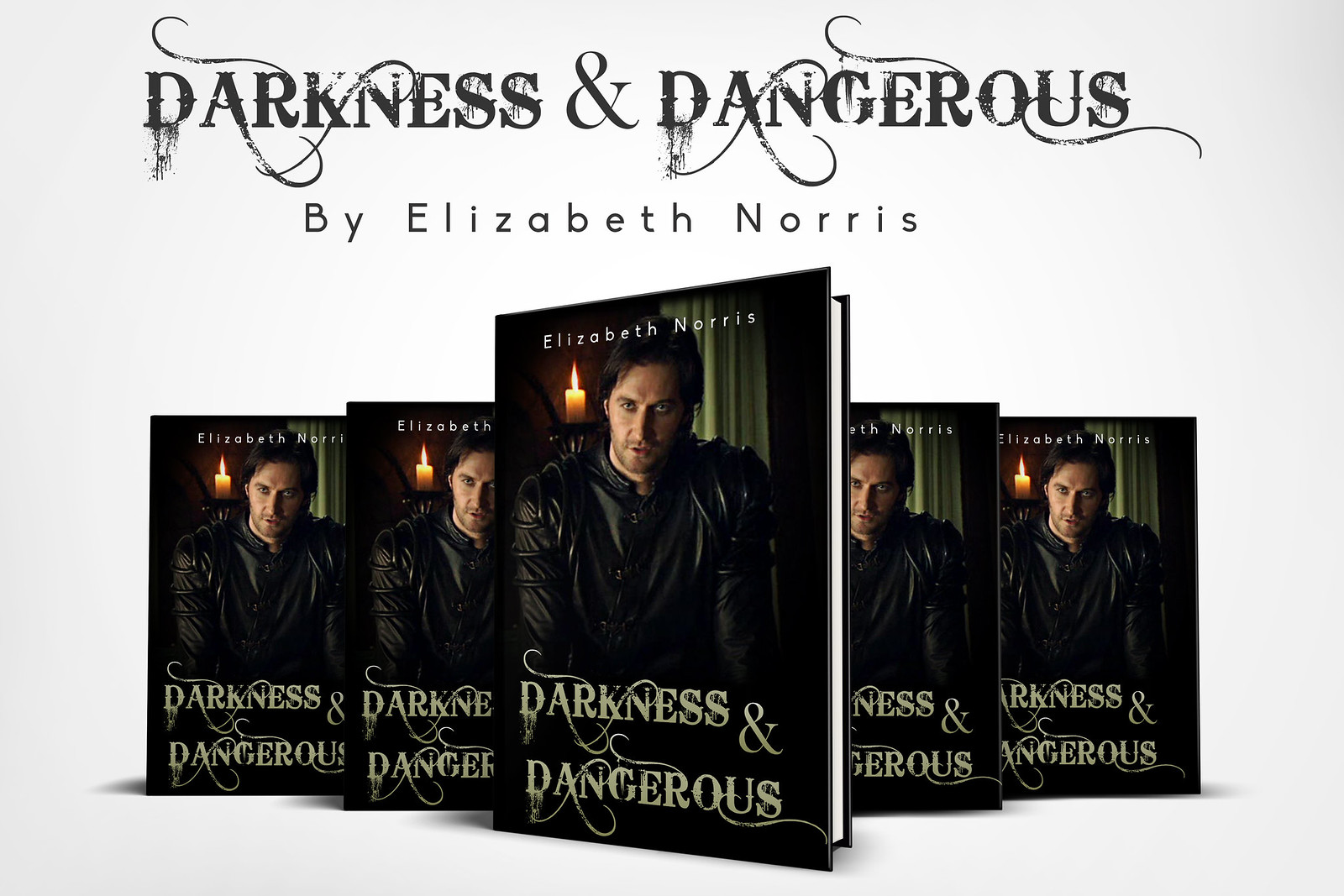This image is an advertisement for a book titled "Darkness and Dangerous" by Elizabeth Norris. Set against a light gray background, the composition features five identical book covers arranged in a pyramid shape, all facing the camera. The focal point is a larger book front and center, with four smaller copies behind it. Each cover has a black backdrop and displays an ominous-looking man in his 30s with dark brown hair, wearing a black leather jacket and a black t-shirt. A burning candle is visible over his right shoulder in the upper left corner of the cover, adding to the eerie atmosphere. The top of each book cover is adorned with the author's name, Elizabeth Norris, in white letters, while the bottom features the title, "Darkness and Dangerous," in an intricate, medieval-style font with swirling scrolls. Above the books, the same text appears in black letters against the white background, with "Elizabeth Norris" written underneath in smaller, dark print.